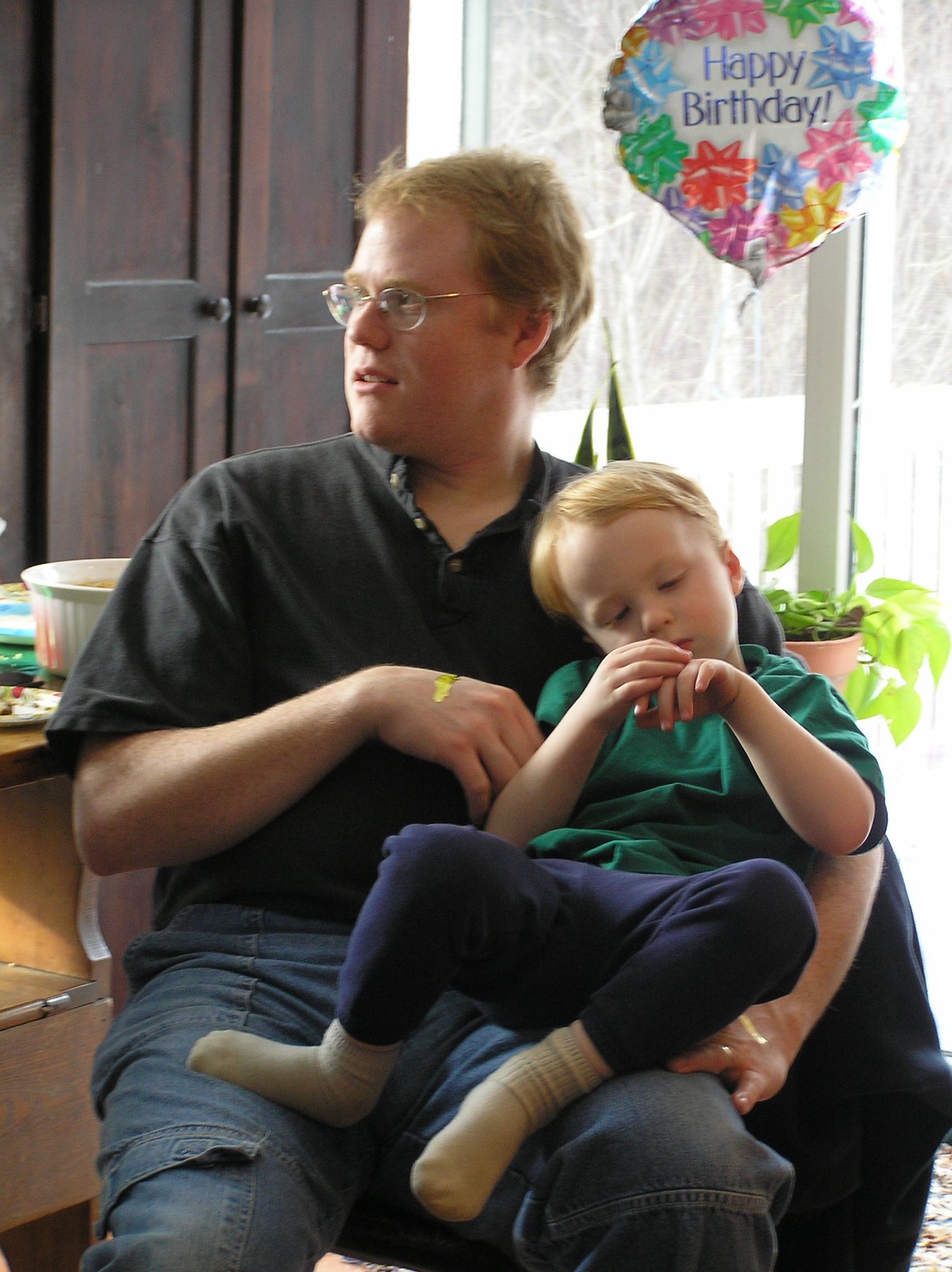A man with blonde, almost reddish hair, and wearing glasses, sits in a chair dressed in a black shirt and blue jeans. He holds a blonde-haired child on his lap, who is wearing a green shirt, blue sweatpants, and white socks. The man has stickers on the back of his hand. In the background, there is a dark walnut cabinet with doors, a potted plant positioned behind the child’s head, and a sliding glass door revealing an outdoor white porch area with bare trees. In the upper right corner, a "Happy Birthday" balloon with pink, blue, red, and green ribbons is visible. Additionally, a table with a casserole dish and a white tablecloth can be seen in the room.